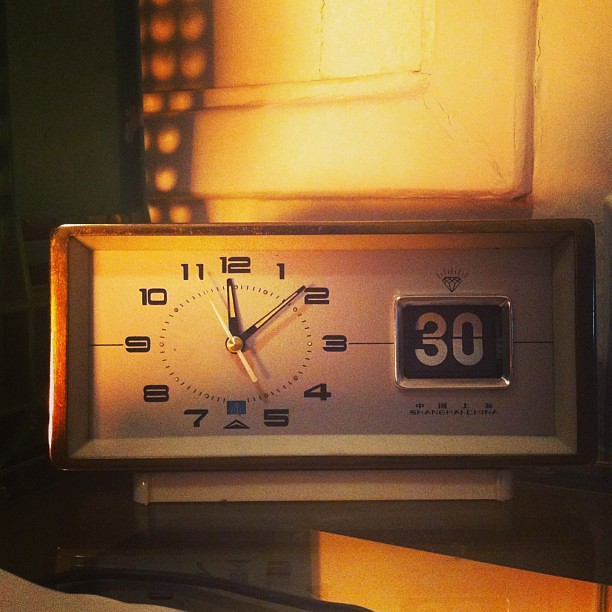This close-up photograph captures a vintage rectangular alarm clock with a polished silver exterior against a stark white background. Positioned on the left side of the frame, the clock features bold, black numerals and distinct black hour and minute hands with white centers, while the seconds hand is entirely white. The time displayed on the clock is 12:09, with the seconds hand pointing at the 11 marker. On the right side, a separate metal square insert is visible, bearing a black background and white numerals at the 30-second mark. Below these numerals, the text "Shanghai, China" is inscribed, and above it, an illustration of a diamond with radiating lines suggests a sparkling effect. The lighting indicates that the photograph was taken in the afternoon, with the setting sun casting a warm glow through a nearby window.